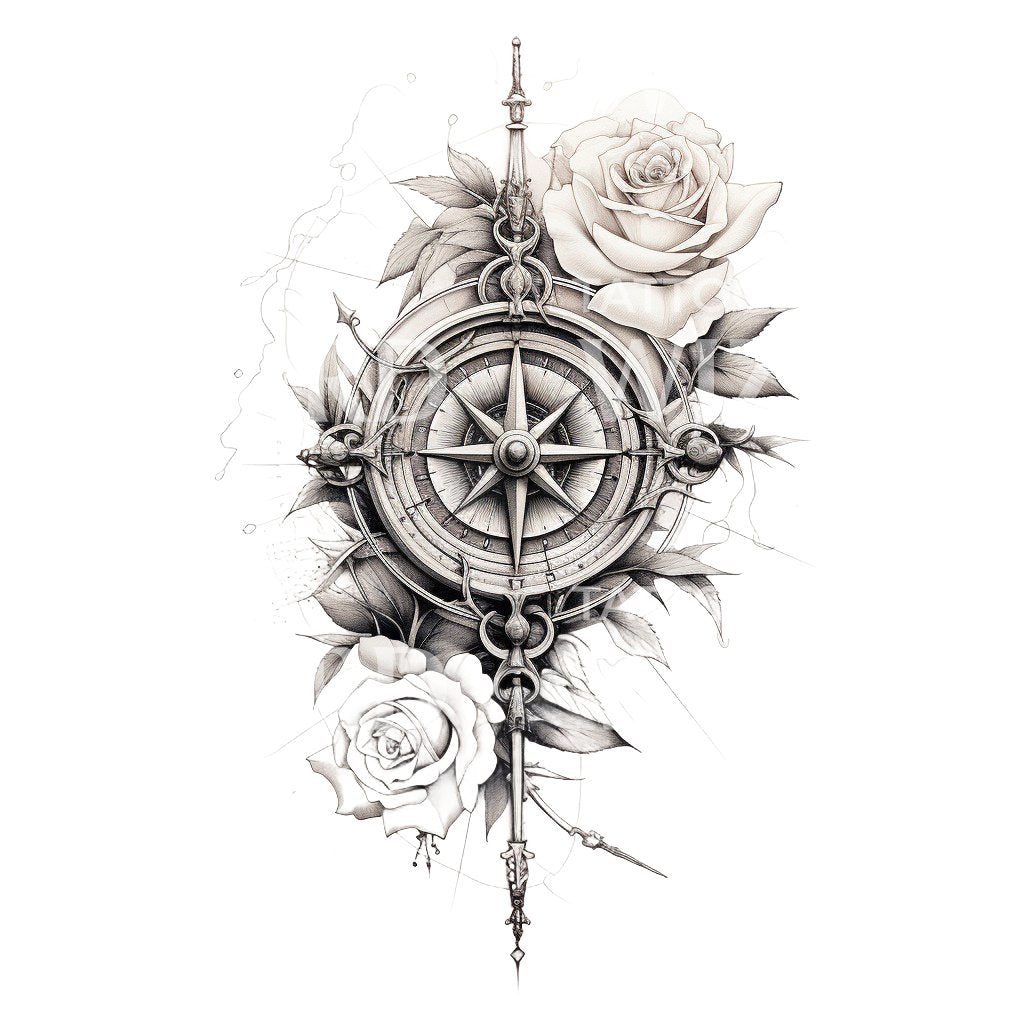This black-and-white illustration, resembling the intricate aesthetic of tattoo art, centers around a detailed compass-like design. The core of the motif features a sun-like object with radiating rays in all directions, overlaid by a multi-ringed structure. Within the central compass, an eight-pointed star dominates, with the cardinal points—north, south, east, and west—distinctly elongated compared to the shorter diagonal points. The compass is adorned with decorative stems extending from the top and bottom. Tick marks frame the dial, adding to its precision. Surrounding this central design are flourishing rose bushes; a fully shaded rose blooms at the top right, complemented by a partially shaded rose at the bottom left. Wispy, delicate lines fill the backdrop, enhancing the overall intricacy of this illustrative piece.